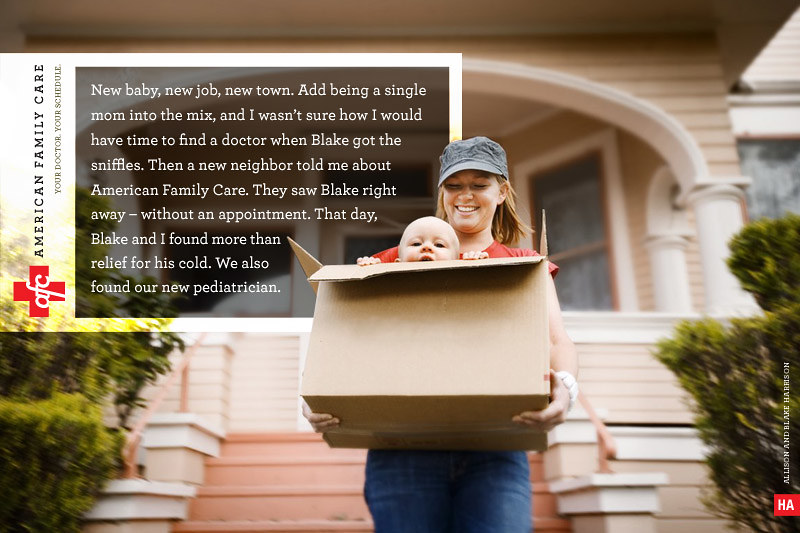In this advertisement for American Family Care, a smiling blonde woman is depicted walking down the steps of a house while carrying a box with a baby peeking out. The mother, wearing a gray hat, a red T-shirt, and blue jeans, looks happily at her child, named Blake. Text on the left side of the image features a red cross with "AFC" along with "American Family Care" and their slogan, "your doctor, your schedule." The accompanying narrative reads: "New baby, new job, new town. Add being a single mom into the mix, and I wasn't sure how I would have time to find a doctor when Blake got the sniffles. Then a new neighbor told me about American Family Care. They saw Blake right away without an appointment. That day, Blake and I found more than relief for his cold; we also found a new pediatrician." This detailed advertisement underscores the convenience and accessibility of American Family Care for busy single parents.